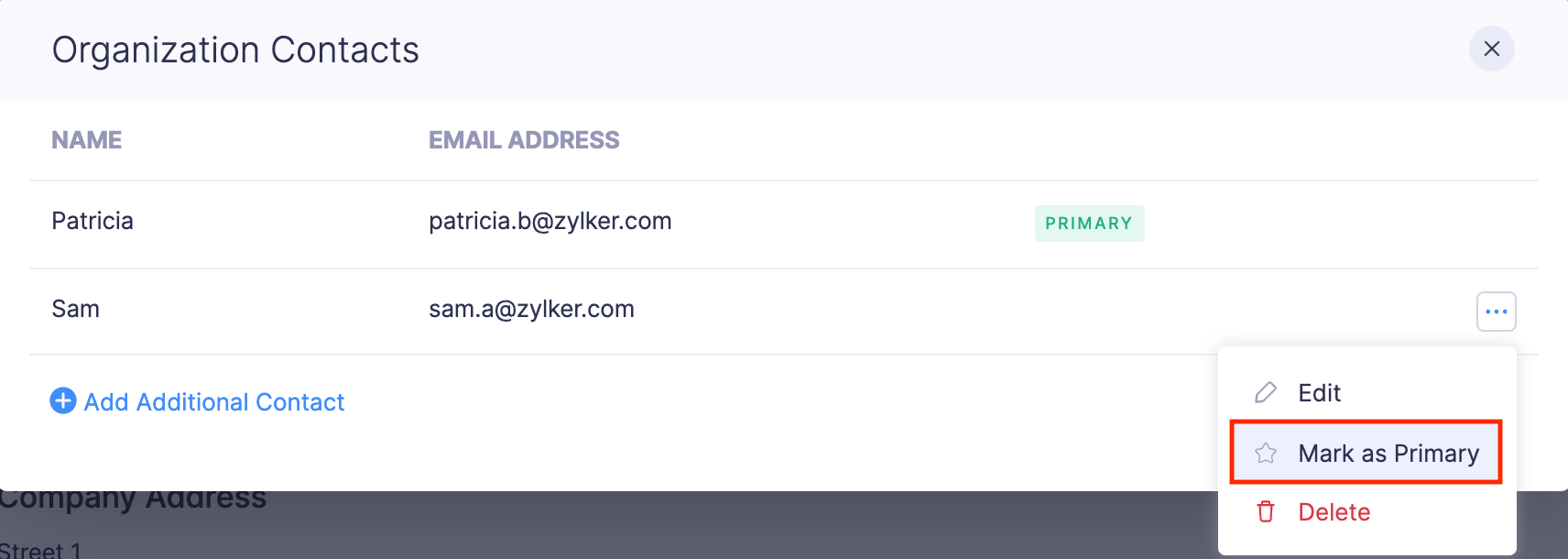The image depicts a digital screenshot of a page titled "Organization Contacts." The title is displayed within a faint, light gray rectangle at the top of the page. To the right of this title is an 'X' icon, which presumably allows the user to close the page.

Beneath the title, the page lists contact names and their corresponding email addresses. The first listed contact is "Patricia," whose email address is Patricia.b@Zilker.com. This contact is marked as "Primary" just below her email address. The second contact on the list is "Sam," with the email address Sam.a@Zilker.com.

Adjacent to the email addresses, there is a horizontal box containing three blue dots, likely indicating additional menu options. Beneath the contact list, a plus sign accompanied by the text "Add Additional Contact" allows the user to add more contacts.

At the bottom of the page is a gray rectangle spanning the width of the screen, with a white box situated on the right corner containing the options "Edit," "Mark as Primary," and "Delete." A red rectangular outline highlights the "Mark as Primary" option, drawing attention to it.